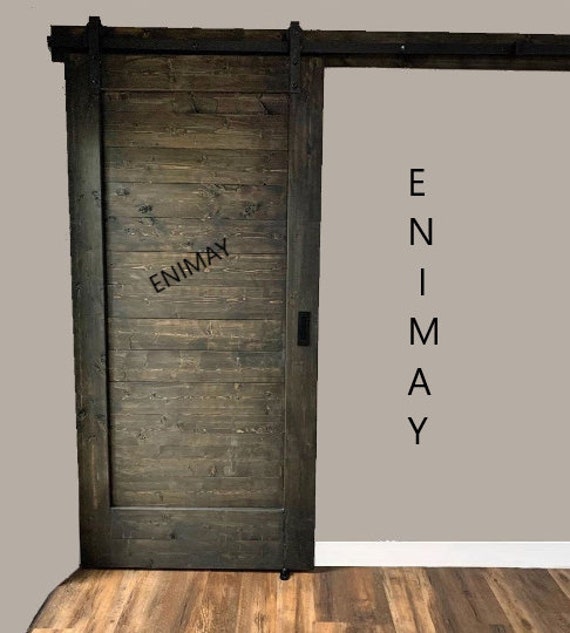The image features a weathered, dark brown sliding wooden door with horizontal wood slats, mounted on a wood rail with black hardware. The door, which has vertical edges and a horizontal piece at the bottom, reveals signs of age, exhibiting a shabby chic aesthetic with visible imperfections. It rests against a gray wall with white trim at the base. The wooden floor beneath the door is a lighter, well-maintained wood. The door and the adjacent digital wall both display the text "N.E.M.A." running vertically in black font. The wall itself, primarily a solid brown-gray color, contrasts with the realistic texture of the wooden elements.